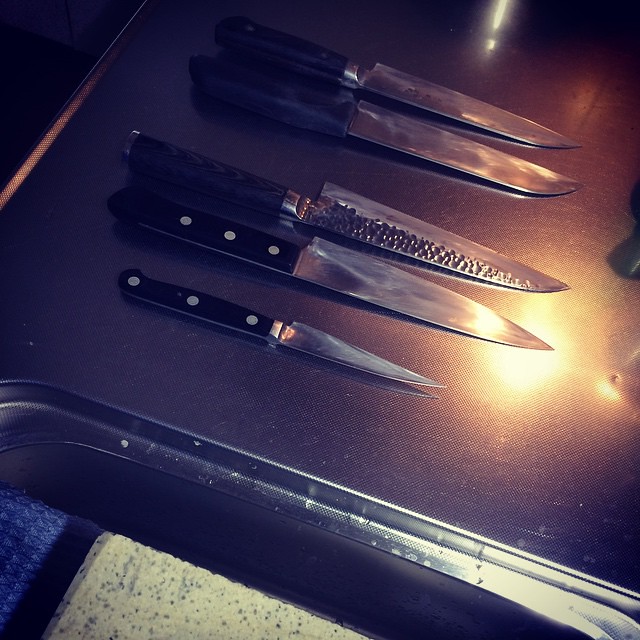This photograph vividly captures five kitchen knives carefully laid out on a gleaming, dark-hued countertop, presumably black or dark blue, next to a chrome sink. A bright light above the sink casts reflections off the metallic surfaces, creating a glowing effect on the scene. Draped over the oven's handle in the background are a blue towel and a white towel, adding a touch of color.

Each knife is arranged horizontally with blades pointing to the right, revealing their sharp, silver edges and black handles. Notably, the middle knife sports a unique hammered metal texture on the non-cutting side of the blade. The remaining knives are of varying sizes and features, with the two knives at the bottom displaying three silver rivets on their black handles.

Within the sink area, partially visible, are several objects including a white item, a blue item, and possibly a sponge, hinting at recent kitchen activities. The overall ambient light is dim, but the central light's yellowish hue prominently illuminates the knives and creates a subtle, reflective glow on the countertop, underscoring the knives' sharpness and well-worn appearance.